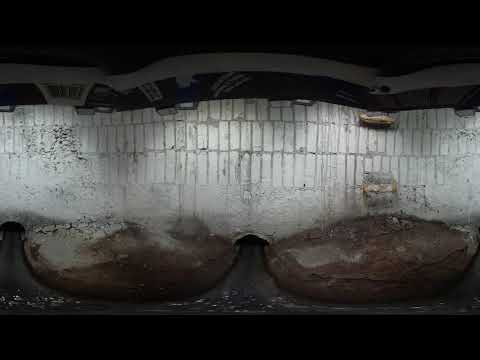The image depicts a distorted, panoramic view of a weathered, gray brick wall with vertical bricks. The surface of the wall shows significant wear, particularly on the left side and bottom, where the texture is rough and worn. The image is in low quality and appears to be taken through a water-streaked or sud-covered window, possibly suggesting the camera is inside a vehicle, like during a car wash. The ground in front of the wall is very dark gray, almost black, with two distinct half-circle mounds of dark gray gravel or dirt. There are drainage canals or holes where the wall meets the ground, one of which is in the middle of the image, and another on the left side, aligning with the half circles. The top and bottom of the image feature black stripes, adding to the distorted perspective. The overall scene has a murky, grimy atmosphere with flowing water and a tunnel-like appearance, contributing to the complex setting of the distorted panoramic view.